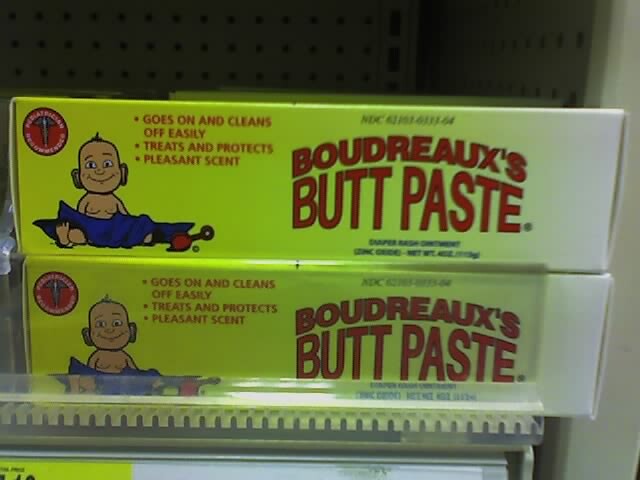This photograph captures two identical packages of "Boudreaux's Butt Paste" stacked on a store shelf. Each package features a cartoon image of a baby with large ears, smiling and wrapped in a blue blanket. A red rattle lies beside the baby. On the top left corner, there's a red circle with small unreadable text. Below the baby, three bullet points in red text detail the product's benefits: "Goes on and cleans off easily," "Treats and protects," and "Pleasant scent." The background transitions from light green to white, and the right side prominently displays the product name. Yellow price labels are partially visible below the packages. The scene includes a black space above the boxes and a white wall to the right.